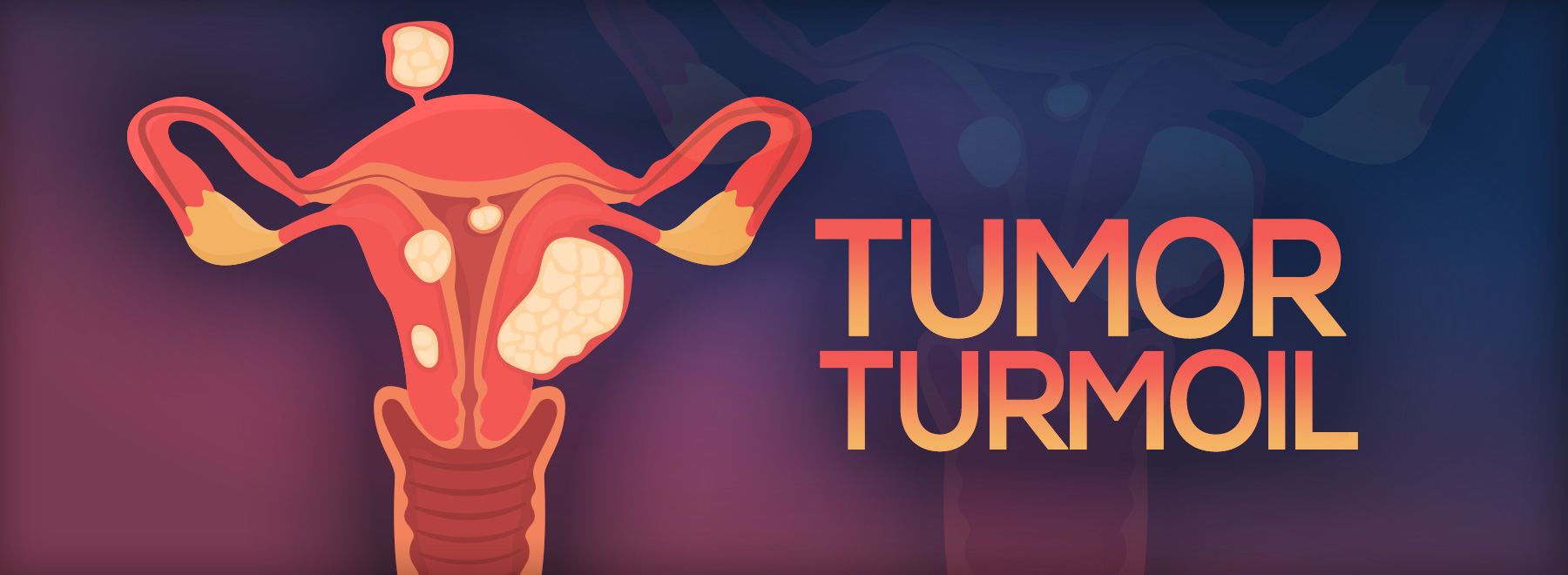The image features an anatomically detailed drawing of a woman's reproductive organs, prominently displaying the fallopian tubes, ovaries, and uterus. The structure is illustrated using shades of orange, darker orange, yellow, and red. Large white masses, identified as tumors or cysts, are dispersed throughout the reproductive system; one is located inside the cervix, while others are embedded in the walls of the uterus and at the top near a fleshy, reddish-pink part. The right side of the image has a dark purple to bluish-purple gradient background, with the bold words "Tumor Turmoil" written in a red, yellow, and orange gradient lettering. The illustration within the image highlights the intrusion of these tumors or cysts in the reproductive organs, emphasizing the pathological conditions depicted.